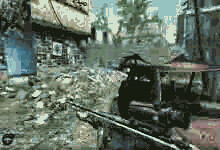The image is a very low-quality, small-sized screenshot, possibly from a first-person shooter video game. Despite being highly distorted and blurred, certain details are discernible. The perspective is from a first-person view, with the player character wielding a machine gun. Dominating the foreground is a bombed building reduced to rubble, with the debris scattered on the ground. To the right, the charred, rusted frame of a car is visible. The backdrop features a couple of trees under a mostly clear, cloudy sky. While the overall scene suggests a chaotic urban environment ravaged by an explosion, it’s challenging to distinguish finer details due to the image's poor resolution and minimal size.